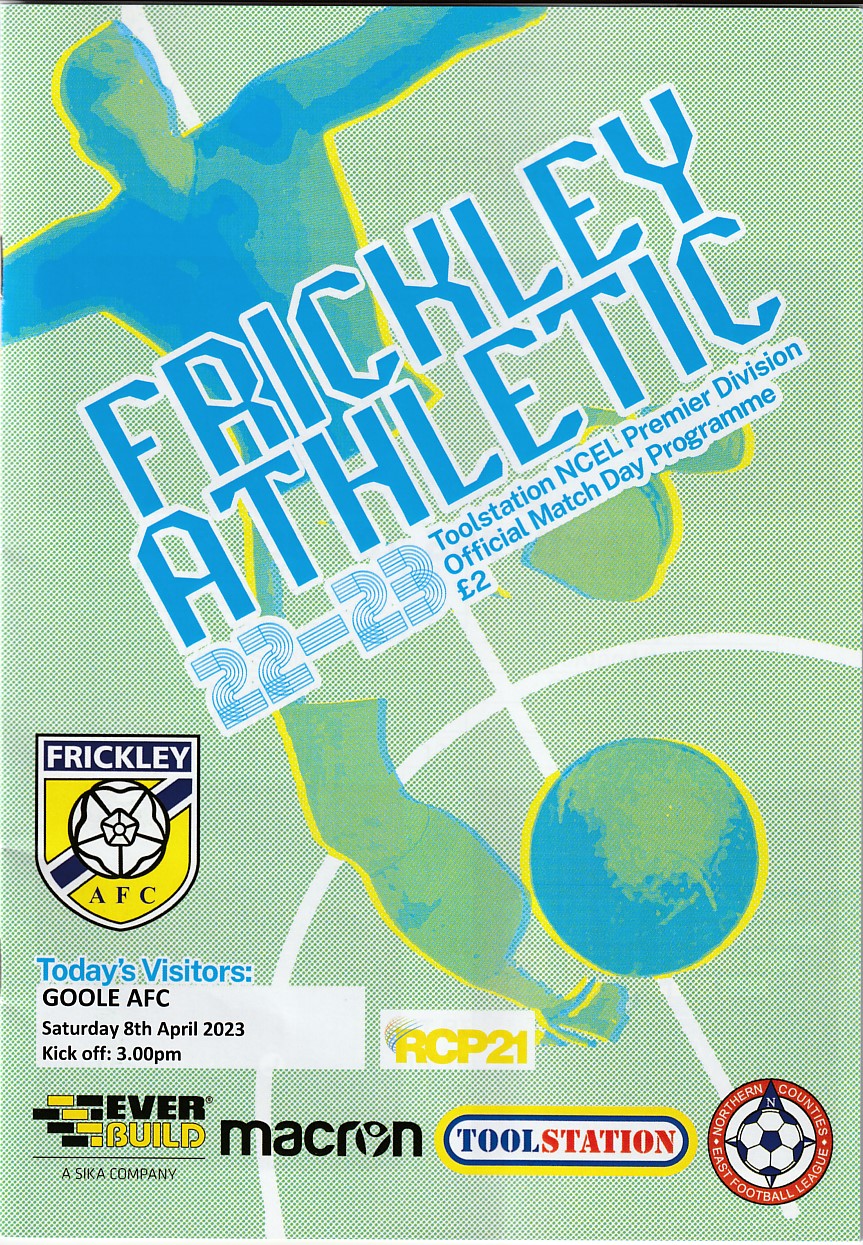This detailed poster provides extensive information about a soccer event hosted by Frickley Athletic. Against a light green background, there is a dynamic silhouette of a player, shaded in blue and green, poised to kick a soccer ball that is below his lifted left foot. Accentuating this action, the silhouette is highlighted with a yellow border. 

The top section of the poster features the team name "Frickley Athletic" in black letters arranged diagonally. Below this, it states "22-23 Tool Station NCEL Premier Division Official Match Day Program Euro 2." On the left side, there's the Frickley AFC logo, a yellow shield with a black soccer ball intersected by a vertical black line, labeled "Frickley" in white text on a black banner. 

Underneath the logo, the poster details the visitor team, reading "Today’s Visitors: Pool AFC" and provides schedule details "Saturday 8th April 2023, Kick-off 3pm." Additionally, sponsor logos are displayed, including Everbuild in black and yellow, Macron with a soccer ball 'O', and the Tool Station logo in blue and red. The bottom left section includes a circular logo with a soccer ball motif. The entire design effectively combines textual information with visual elements to announce the match day clearly and attractively.